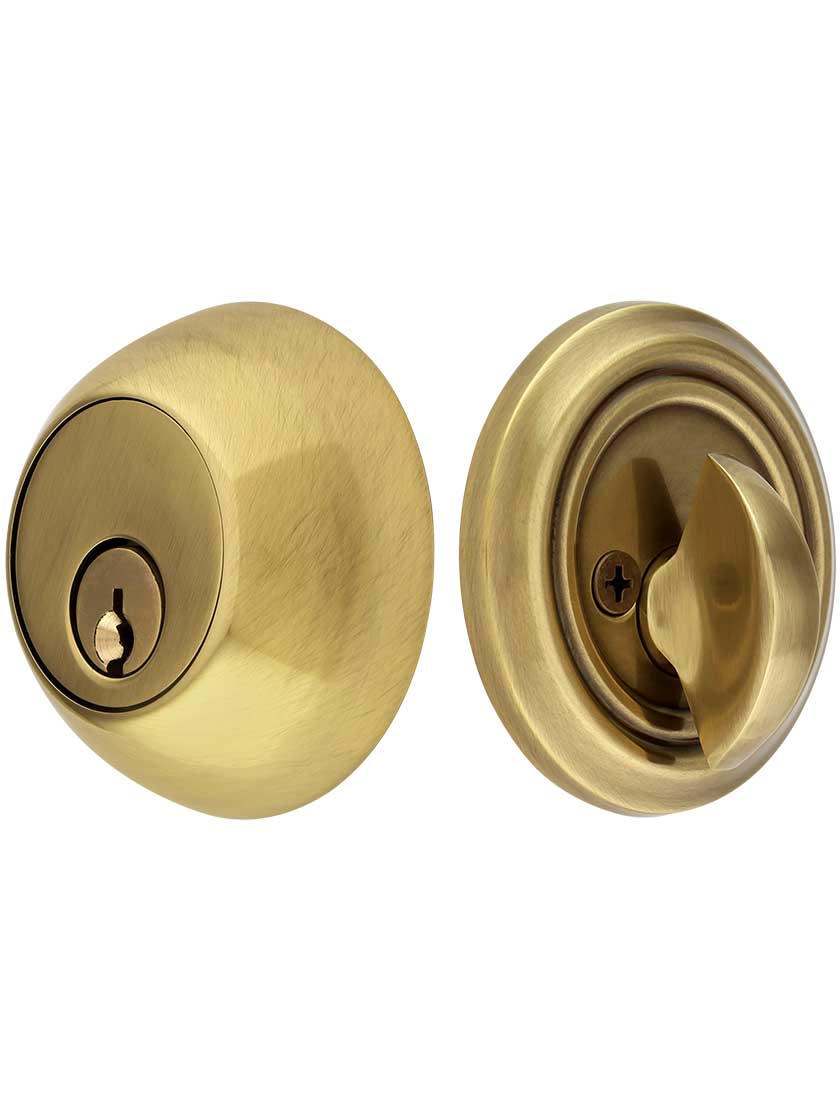The image showcases both sides of a brass door lock against a stark white background, suggestive of a catalog or advertisement. On the left-hand side, the lock's exterior features a shiny brass keyhole, where a key can be inserted and turned. The right-hand side displays the interior mechanism, equipped with a horizontal turning knob for locking and unlocking from inside. Notably, next to the knob on the right side is a visible Phillips head screw. The depicted lock is highly detailed, with a finish so polished that it is difficult to distinguish whether it is a photograph or an exceptionally realistic illustration. Both sides of the lock are positioned at a slight angle, with the key side oriented 45 degrees to the left and the knob side 45 degrees to the right, emphasizing their dimensional quality.